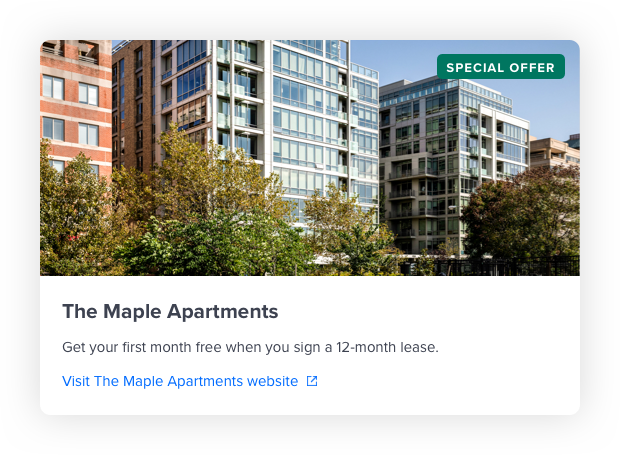The image depicts a cluster of apartment buildings, prominently showcasing two tall, gray structures with numerous uniform windows. Each window features drawn shades, contributing to a uniform facade. Flanking these buildings, on the left, stands a red brick building, and to the right, there is a brown brick building. The forefront of the image is adorned with several trees and a boundary fence, adding a touch of greenery to the urban landscape. 

In the top right-hand corner, a green box with white text announces a "Special Offer." Below the image, a white box contains a caption in black text that reads: "The Maple Apartments. Get your first month free when you sign a 12-month lease." A clickable link to visit The Maple Apartments' website is also provided in blue text.

The height and uniformity of the windows in the gray buildings suggest impressive, towering structures, giving a sense of the architectural scale within the image.